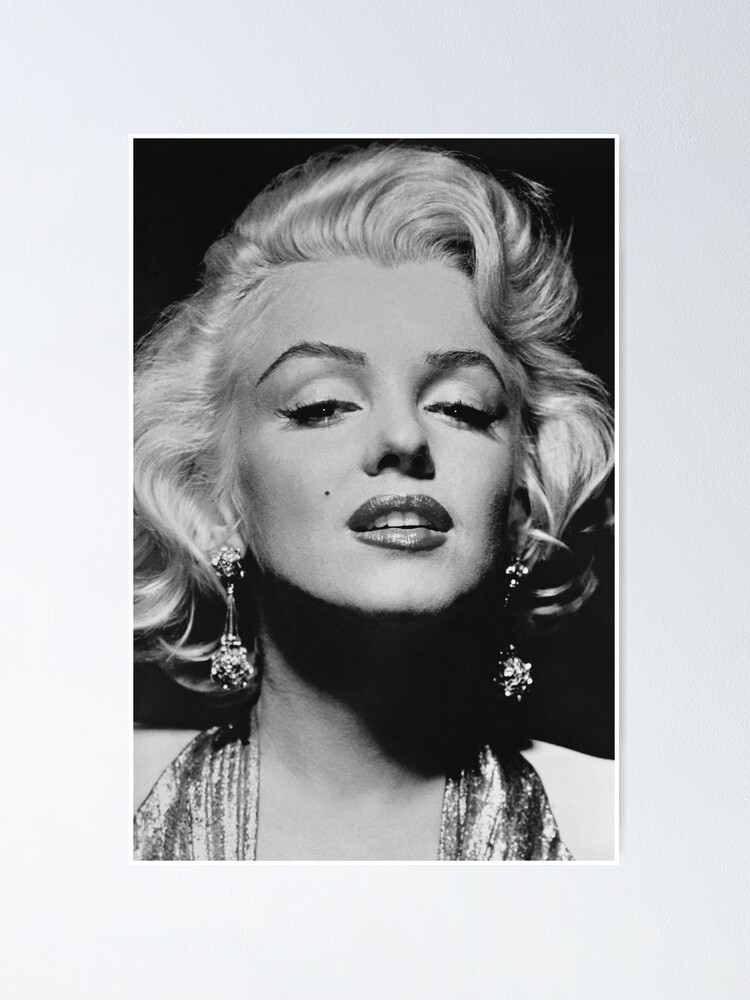This is a vertical black-and-white photograph featuring Marilyn Monroe in a classic headshot against a pitch-black background. The image is framed by a thin white border and encased in a thicker gray mat, giving it a polished presentation. Marilyn's signature short blonde hair, styled in voluminous waves with a swoopy side part, frames her face. Her makeup is distinct, with thick mascara, eyeliner, and visible lipstick. Her eyes are half-closed, revealing her irises and pupils partially. A characteristic mole is present on the right side of her cheek, while she slightly tilts her chin upward, gazing towards the viewer. She’s adorned in long, dangling chandelier-style earrings that appear shiny and metallic in the black-and-white format. Her outfit, though only partially visible, features sleeveless metallic straps around her collarbones. Most of her neck is enveloped in shadows, adding to the dramatic effect of the photograph.